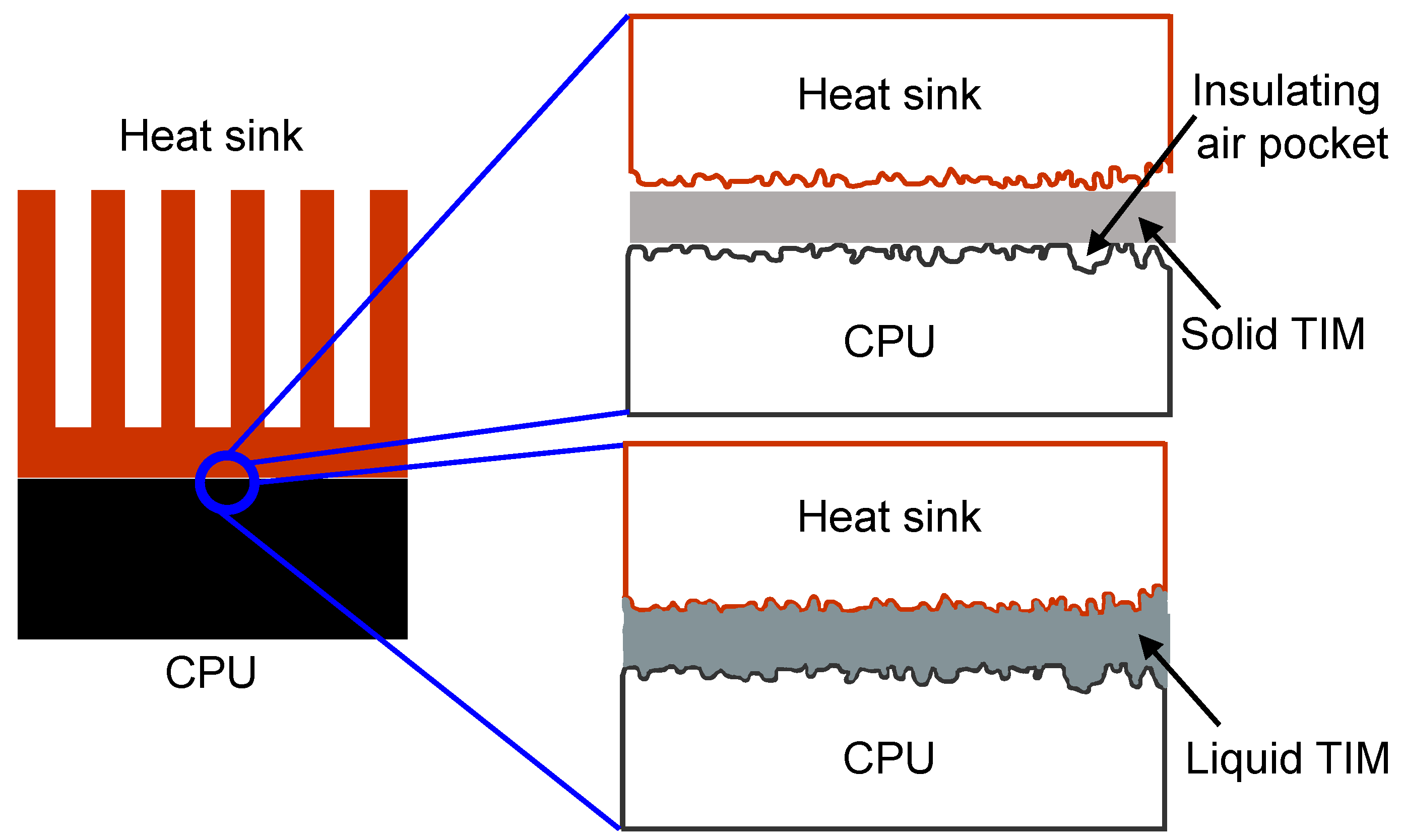The image is a detailed technical infographic illustrating CPU heating elements and their components. The diagram, which is in landscape orientation, presents a series of interconnected elements starting from the left. At the far left, there is a black horizontal rectangle labeled "CPU". On top of this rectangle is a red object resembling an inverted pitchfork, labeled "Heat Sink". 

Central to the infographic is a blue circle from which four lines radiate to different sections of the diagram. The first section at the top showcases a red rectangle labeled "Heat Sink", beneath which is a gray bar marked as "Solid TIM" (Thermal Interface Material), indicating a solid thermal interface. Directly below this, an arrow points to another section labeled "Insulating Air Pocket", identified by a squiggly line pattern, signifying an air pocket that provides insulation. 

The second section down features another red rectangle also labeled "Heat Sink". Below it is a gray area termed "Liquid TIM", suggesting a liquid thermal interface material. The final section at the bottom displays another black rectangle labeled "CPU". 

Overall, this infographic provides a comprehensive, color-coded, and text-labeled breakdown of the heat management components associated with a CPU, delineating the roles and positions of various thermal interface materials and heat sinks in a systematic, scientific illustration style.